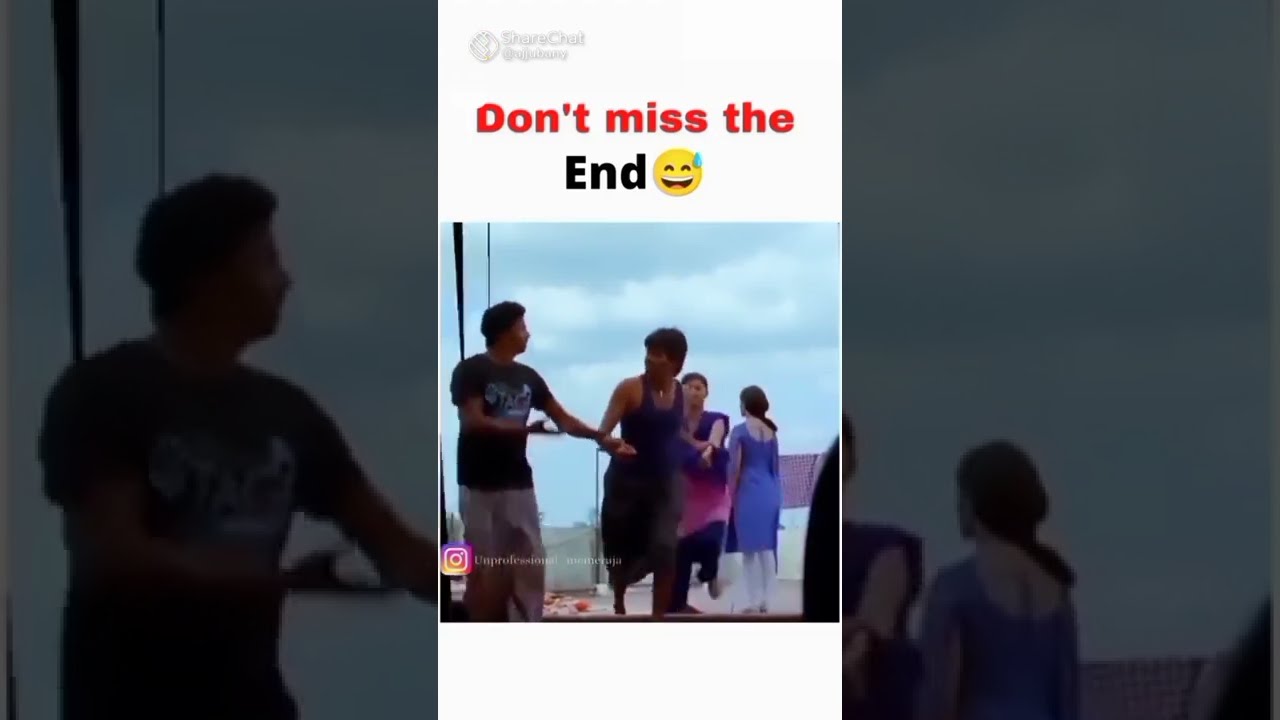This photograph captures a lively outdoor scene featuring four individuals—three women and one man—under a blue sky with scattered clouds. In the foreground, the man, dressed in a black t-shirt and gray pants, is animatedly raising his right arm while clasping the right arm of a woman in a long purple dress with his left hand. Behind them, two women engage in conversation; one sports a long blue dress, while the other wears a long black and purple dress. Intricately, the image is set within a vertical cell phone frame, bordered by white with text at the top and bottom. The top text in red reads "Don't miss the," while the bottom text in black says "end," accompanied by a smiling emoji with a tear. The faded and zoomed-in background mirrors the main image, focusing on the man in the foreground and the woman in the blue dress. An Instagram icon is subtly visible in the lower left corner, adding a contemporary touch to this candid moment that hints at a lively gathering, possibly a karaoke session.